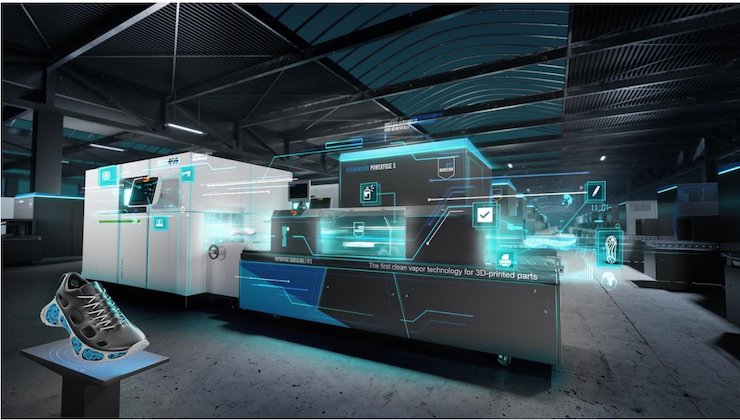In the image, a large, futuristic factory or warehouse is depicted, composed mainly of corrugated metal and glass. The floor is constructed of gray concrete, and the ceiling is lined with black panels featuring dark teal accents. A central, half-domed glass channel runs along the middle, allowing a view of a dark blue sky above. The space is filled with numerous rows of white and black machinery with blue trim, extending into the background. 

To the left, among these machines, is a white square machine and a rectangular silver machine with a squared box on top. Floating CGI digital display screens are positioned in front of these machines, one of which reads "the first clean vapor technology for 3D printed parts."

In the foreground is a striking anomaly: a running shoe mounted on a pedestal. The shoe, gray in color with blue lace strings and resting on a wide sole adorned with blue and white cutouts, sits atop a black podium with a blue top, drawing attention as the single piece of footwear stands conspicuously out of place amidst the high-tech environment.